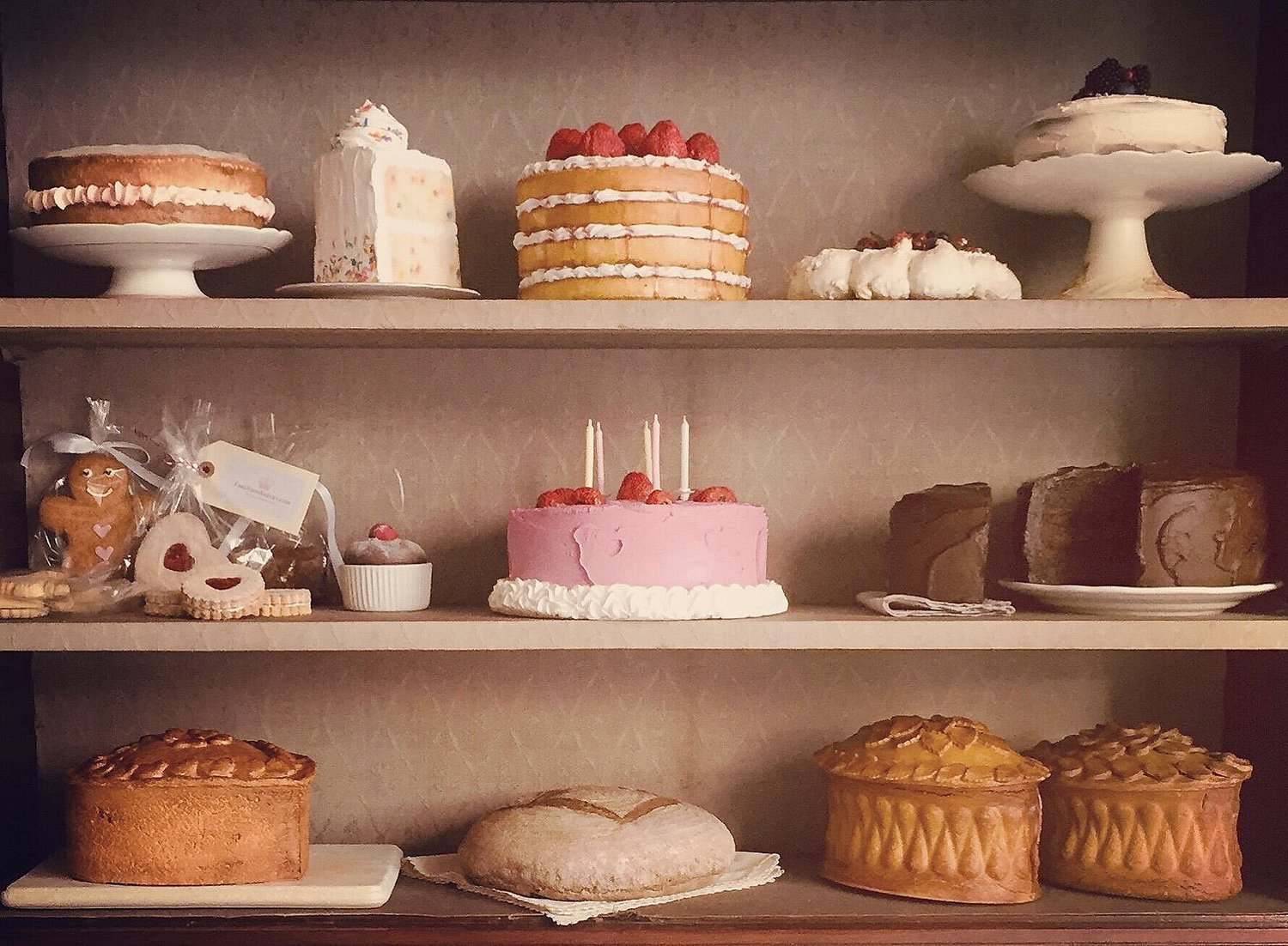This image depicts a variety of pastries and baked goods artfully arranged on three wooden shelves in what appears to be a coffee shop or bakery. The bottom shelf is a dark brown, while the middle and top shelves are light brown. On the top shelf, a brown cake with white inner cream sits on a white platter, flanked by a large white double-confetti cake. Nearby, a four-layered strawberry and cream cake garnished with strawberries and five white candles is prominently displayed. Additionally, there is a small white fluffy cake on a tall cake stand, and a white frosted cake with berries.

The middle shelf showcases a diverse selection of treats, including a pink frosted cake with a quarter cut out and a chocolate cake. Some pastries are wrapped in plastic, resembling gingerbread men, along with cupcakes and plastic-wrapped baked goods.

On the bottom shelf, a selection of fancy molded breads lies, all looking delicious but indulgent. The overall presentation of these confections suggests a tempting assortment that would be a delight for any dessert lover.